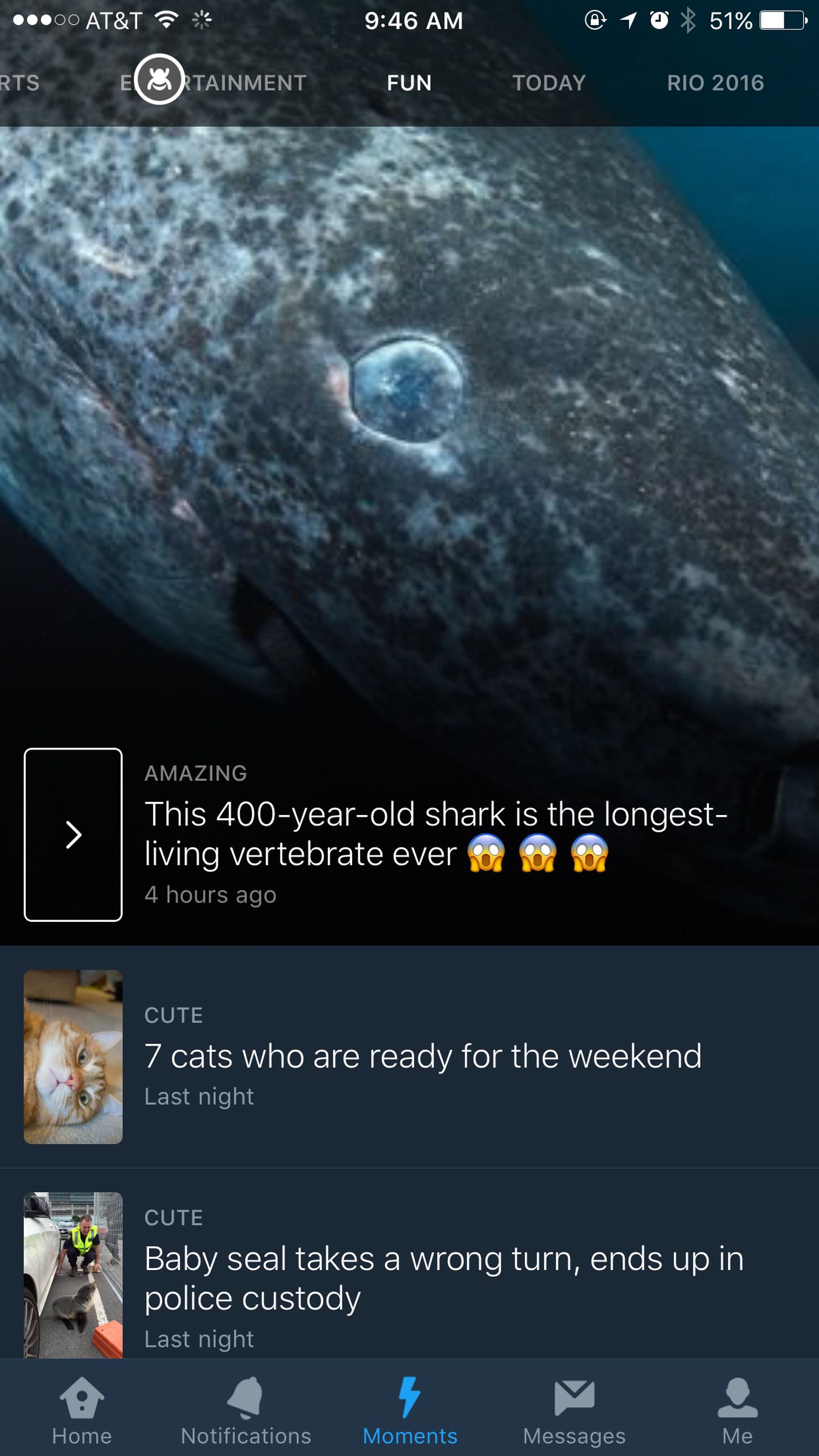### Detailed Descriptive Caption:

A screenshot from a mobile device displays a selection of news articles under the "Fun" category. Dominating the screen is a large image of an ancient shark, corresponding to a headline that reads, "This 400-year-old shark is the longest living vertebrate ever," posted four hours ago. The screenshot captures additional content, including articles in the "Cute" section, with headlines such as "Seven cats who are ready for the weekend," and "Baby seal takes a wrong turn, ends up in police custody."

At the top of the screen, indicators show the device is connected to AT&T's network with both Wi-Fi and cell signal strength visible. The time reads 9:46 a.m., and the battery is at 51%. The status bar also reveals that alarms are set and the screen is locked.

At the bottom of the screen, five navigation options—Home, Notifications, Moments, Messages, and Me—are visible, with "Moments" currently selected. This screenshot provides a detailed glimpse into the device's interface and the user's engagement with diverse and intriguing news content.